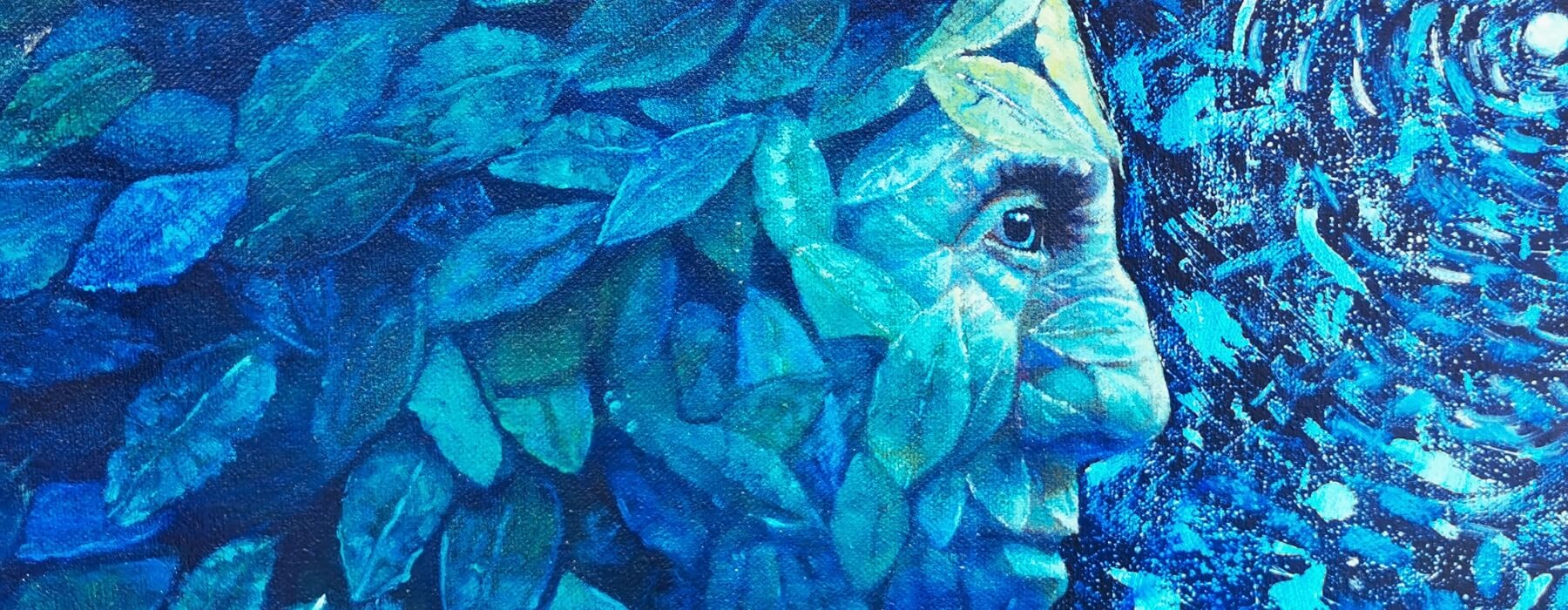The horizontally rectangular image, possibly a painting or colored drawing, features a mature-faced individual of Indian descent subtly blended into a vibrant foliage backdrop. Dominating the left half, the foliage consists of an array of blue leaves, ranging from aqua green to dark navy royal, with some appearing bluish-green or fungal-like in shape. These leaves cascade and partly obscure the individual’s facial features—including his big nose, large blue-ringed eyes, mouth, and cheeks. The person appears to be gazing thoughtfully to the right. To the right of the face, swirling bands of light blue, green, and darker blue or purple colors evoke an underwater scene, populated possibly with fish-like shapes, dust-like white specks, and culminating in a small white sphere in the upper right-hand corner. The entire composition, from the intricate leaf details to the swirling aquatic colors, combines to create a mysterious and ethereal visual experience.